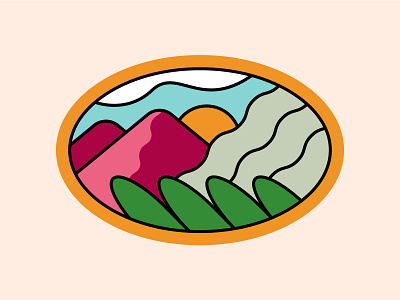The image features a centrally placed, egg-shaped logo outlined in orange, rotated 90 degrees to lie on its side. The background is a gradient of peach to light pink. Inside the logo, simplistic, stained-glass-like designs are outlined in black. On the left side, two red triangular mountains rise up. Nestled between the mountains and the shapes on the right is a small, orange sun without rays, symbolizing sunrise or sunset. Below the mountains, there are four tall, oval green leaves, slightly tilted. On the right side, three wavy light sage green lines represent waves. Above these elements, a section of blue denotes the sky, capped with a few white clouds.